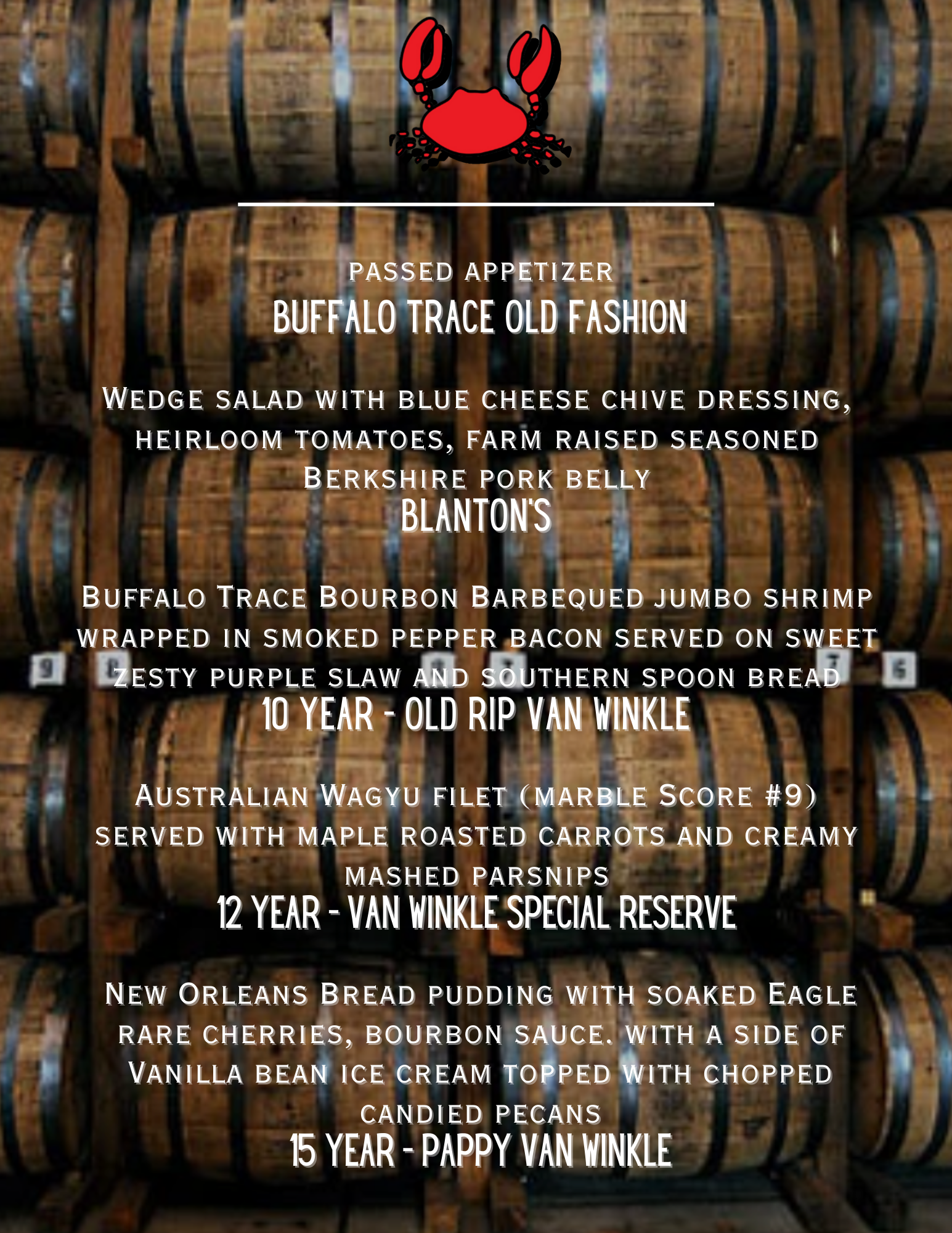The image displays a menu overlaid on a backdrop of stacked whiskey barrels. The barrels, positioned horizontally, reveal partial views of the outermost barrels on the left and right. Each barrel is adorned with six black stripes, including the top and bottom edges. Centered at the upper part of the image is a red cartoon crab. Below the crab, in carefully arranged text, is the menu detailing an array of appetizing dishes.

The menu begins with "Past Appetizers, Buffalo Traced Old Fashioned" followed by a "Wedge Salad with blue cheese, chive dressing, heirloom tomatoes, and farm-raised seasoned Berkshire pork belly" accompanied by "Blantons." Next is the "Buffalo Trace Bourbon Barbecued Jumbo Shrimp wrapped in smoked pepper bacon, served on sweet zesty purple slaw and Southern spoon bread," paired with "10-year-old Rip Van Winkle."

Continuing with the entrees, the menu features "Australian Wagyu Filet, marbled score number 9, served with maple roasted carrots and creamy mashed parsnips," alongside "12-year-old Van Winkle Special Reserve." The final item is a decadent dessert: "New Orleans Bread Pudding with soaked Eagle Rare Cherries, bourbon sauce, a side of vanilla bean ice cream, topped with chopped candied pecans," complemented by "15-year-old Pappy Van Winkle."